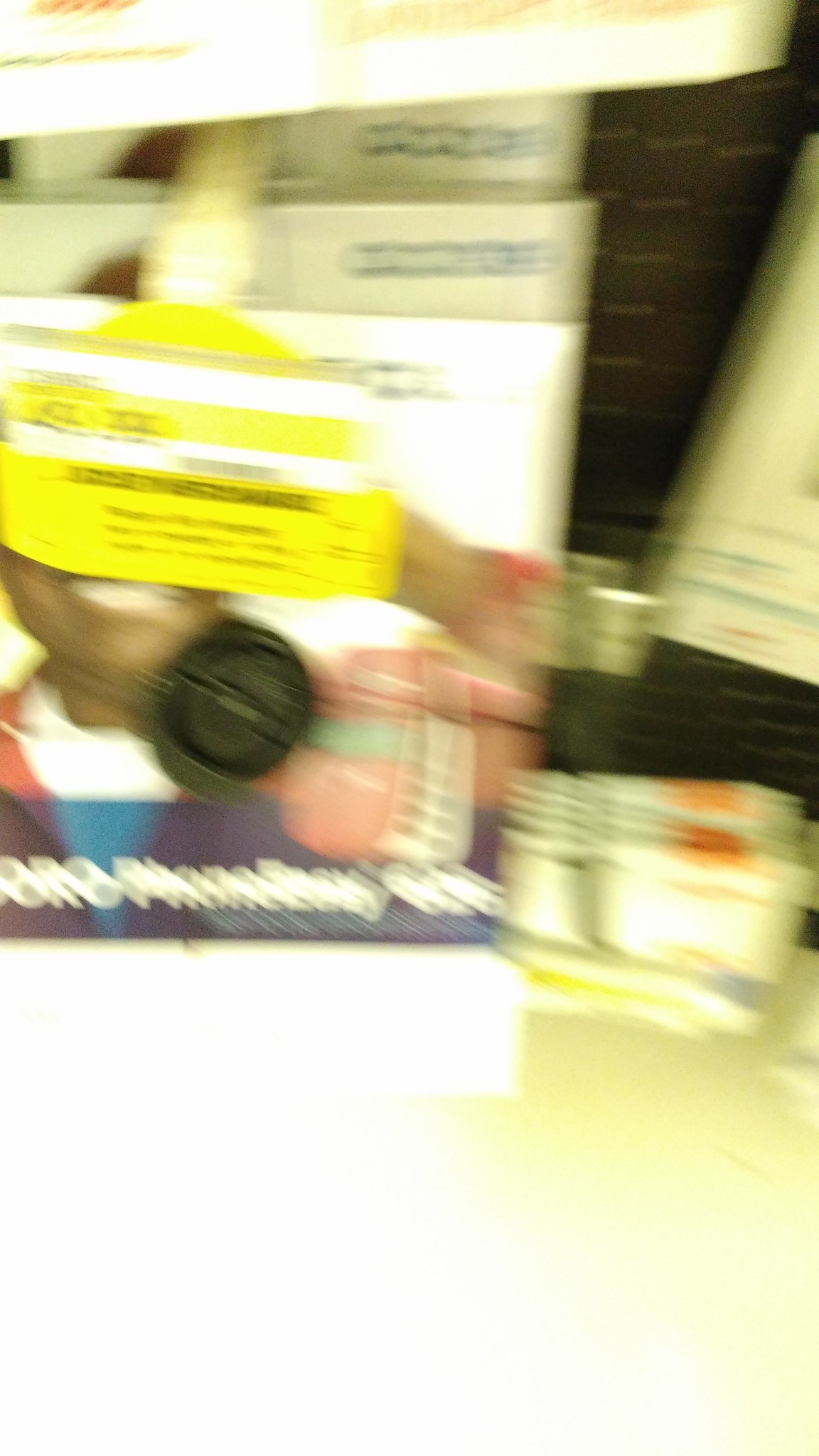The photograph captures an indoor setting, likely within a store, showcasing a shelf laden with various consumer goods which might include magazines or books. The image is notably overexposed, resulting in extremely bright objects that are hard to distinguish due to the glare. Additionally, the photograph suffers from significant motion blur, further obscuring the details of the items present. On one of the items displayed on the shelf, there appears a person's face partially hidden by a yellow label with indecipherable black text. The visible part of the face shows a person with dark skin and strikingly white teeth. The individual is adorned in a multicolored shirt featuring shades of white, red, purple, and blue, and seems to be grasping an unidentified item that is concealed behind the label. The overall effect of the overexposure and blurriness leaves much of the scene indistinct and challenging to interpret clearly.